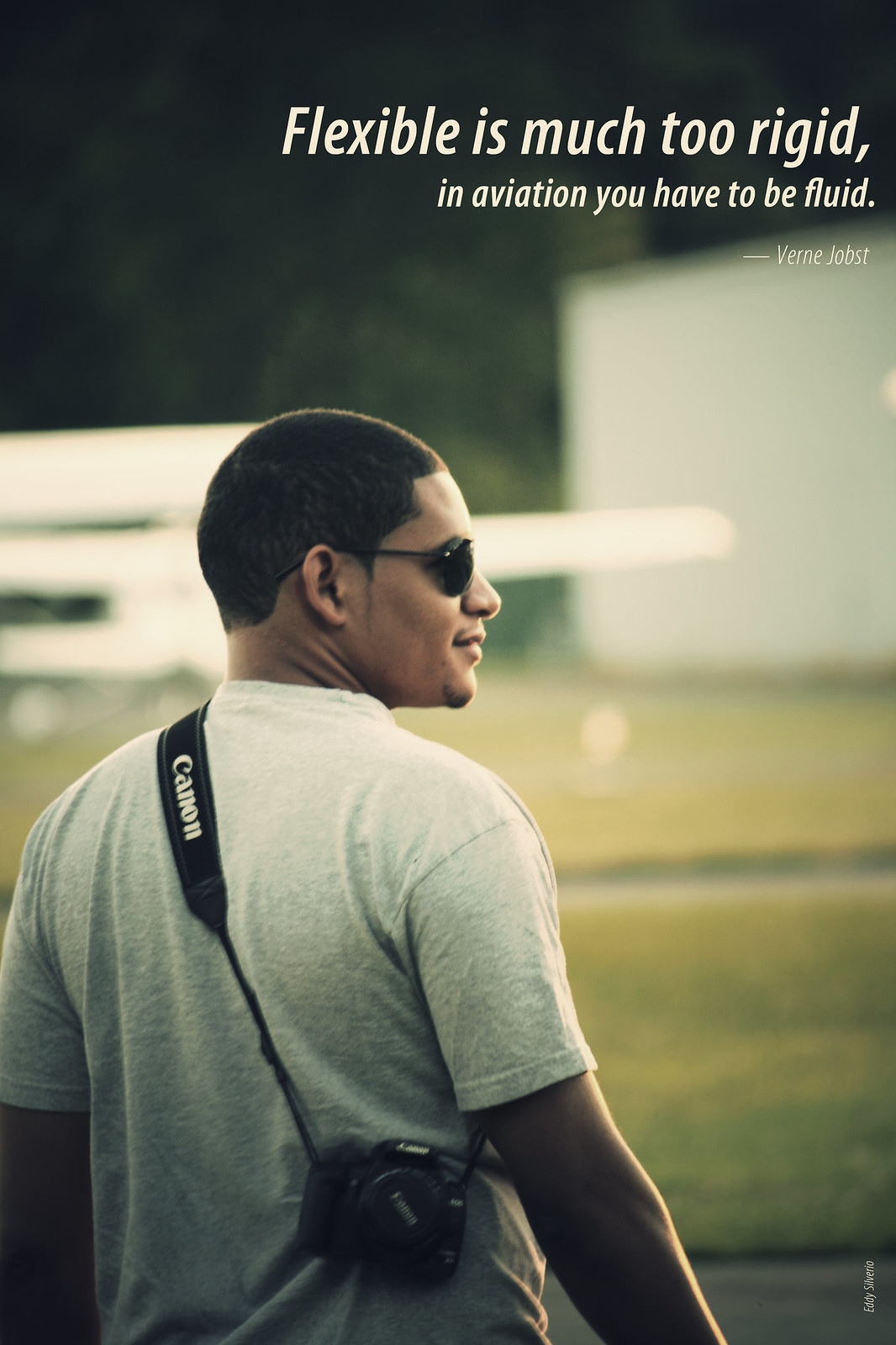**Caption:**
At the top of the photograph, an inspirational quote reads, "Flexible is much too rigid. In aviation, you have to be fluid," attributed to Hyven Verne Jobst. Below the quote, centered at the bottom of the image, a black man stands with his back to the camera, his head turned to the right, revealing his profile. He wears dark black sunglasses, has short black hair, and sports a goatee and mustache. Dressed in a gray shirt, he has a camera with a white "Canon" strap slung over his shoulder, hanging behind his arm. 

The background is heavily out of focus, featuring what appears to be a mix of light green and yellow grass with a couple of pink glares, one intersecting the man's face. Above him, the sky appears dark as though it is night, with some light shining down from an unspecified source. On the upper right of the image, a small white structure is visible, resembling a tiny building. On the left side, there is another indistinct white object that could be bleachers, but the heavy blur makes identification difficult. The photograph captures a contemplative moment, blending the contrast between clarity and ambiguity, much like the quote suggests the necessity of fluidity in aviation and life.